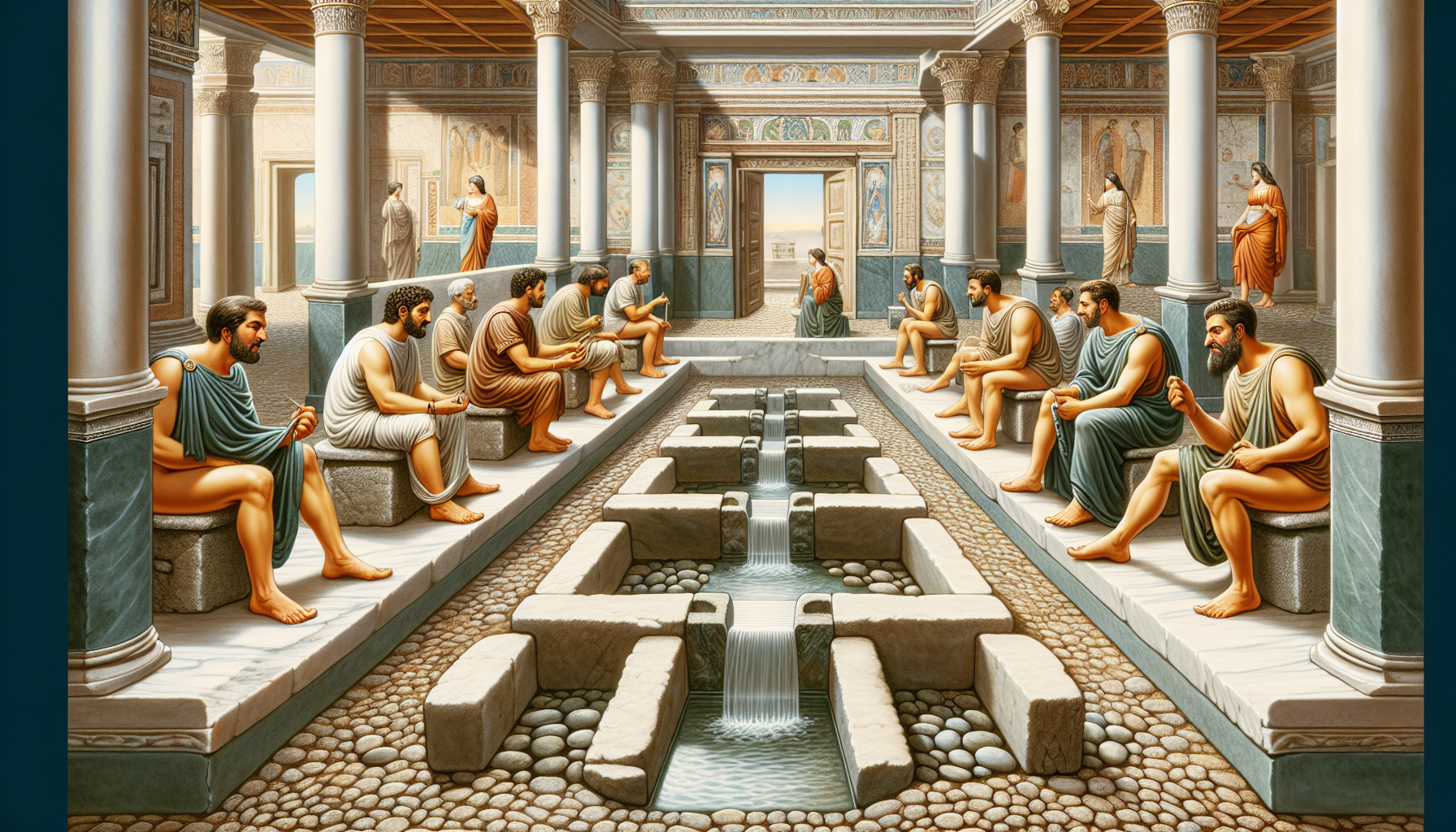This detailed painting depicts an ancient Roman-inspired interior chamber. The scene is richly colored and filled with architectural splendor, featuring numerous white pillars supporting the roof and stone walls adorned with various intricate symbols and designs. 

In the center of the image is a flowing creek that runs the length of the room, accentuated by large, rectangular concrete blocks over which the water cascades. These blocks create a series of U-shaped formations, guiding the water in an artistic manner. 

On each side of the creek, platforms raised slightly above the floor accommodate rows of stone seats. Six men, each with short dark hair, are seated on the left, facing five men on the right. They wear togas in a range of colors including green, white, blue, red, and brown. 

In the background, beyond the men and closer to the open double doors, stands a person in an orange and blue toga, kneeling. Inside this grand chamber, five columns on either side support the structure. Near these columns, additional figures dressed in variously colored robes—white, orange, and blue—appear to be engaged in conversation or observing the scene. 

Altogether, the painting captures an atmosphere of serene order and detailed architectural beauty, combining the elements of classical design with the vivid portrayal of social interactions and structural elegance.